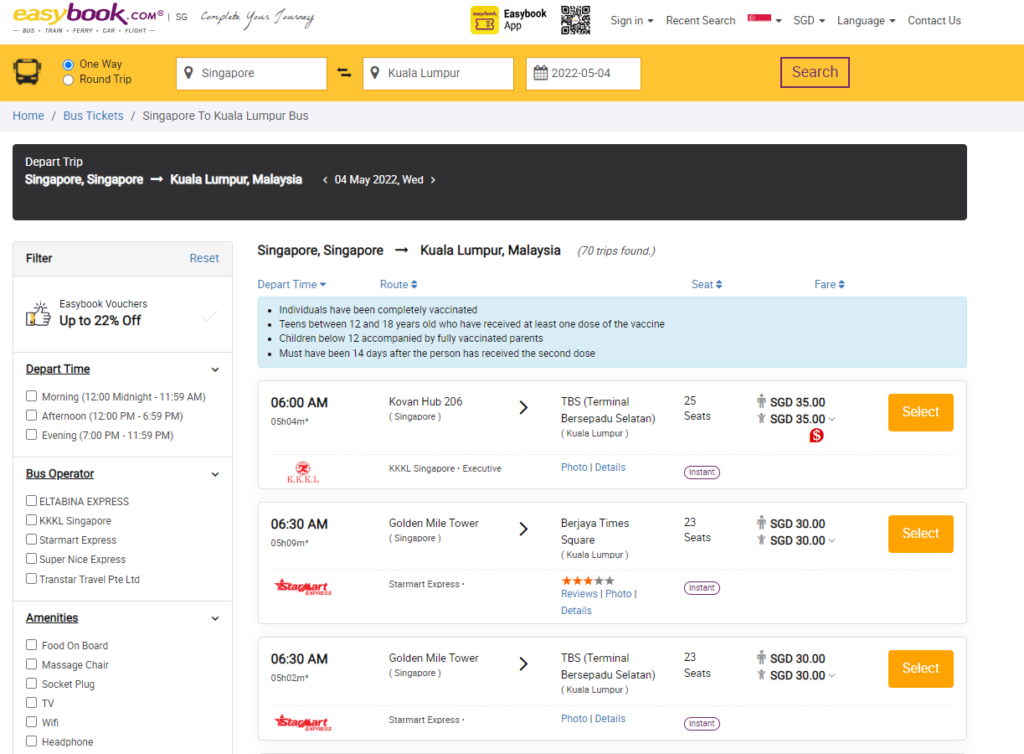The image showcases a computer screen displaying the EasyBook.com website, with all text written in lowercase letters. The word "easy" is highlighted in yellow, while "book" is in bold purple, and "dot com" in a less bold purple, accompanied by a trademark symbol. The tagline "complete your journey" is prominently placed beneath the site’s name.

At the top of the screen, the text "Facebook app" is visible, alongside a QR code designed for easy scanning. Other functional elements like the sign-in option, recent searches, language selection (SGD), and a "contact us" link are also present.

A gold bar stretches across the screen. Just below, there’s an image of a bus, highlighting options for selecting between a one-way or round-trip journey. The displayed choice is a one-way trip from Singapore to Kuala Lumpur, with a date set for May 4, 2022.

Navigational links at the top include "home," "bus tickets," and "Singapore to Kuala Lumpur bus," indicating a short trip. On the left side, there are various filter options for users to save money and choose different operators to narrow their search. The results provide three different bus options, detailing departure times and drop-off locations.

The overall purpose of the webpage is to assist users searching for bus tickets specifically for travel from Singapore to Kuala Lumpur.